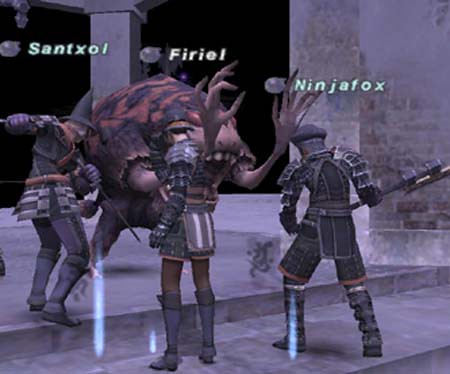The digitally created image, likely a screenshot of a video game, depicts a dark-toned scene with three armored knights standing on wide marble steps in a grand setting featuring marble columns and a brick wall in the upper right corner. The knights, each equipped with distinct weapons—one with a sword, another with an axe—are ready to engage in battle with a blob-like mythical creature with short, stubby hands raised menacingly towards them. Above each knight, white text identifies them as SandXOL on the left, Furiel in the center, and NinjaFox on the right, indicating their player names.